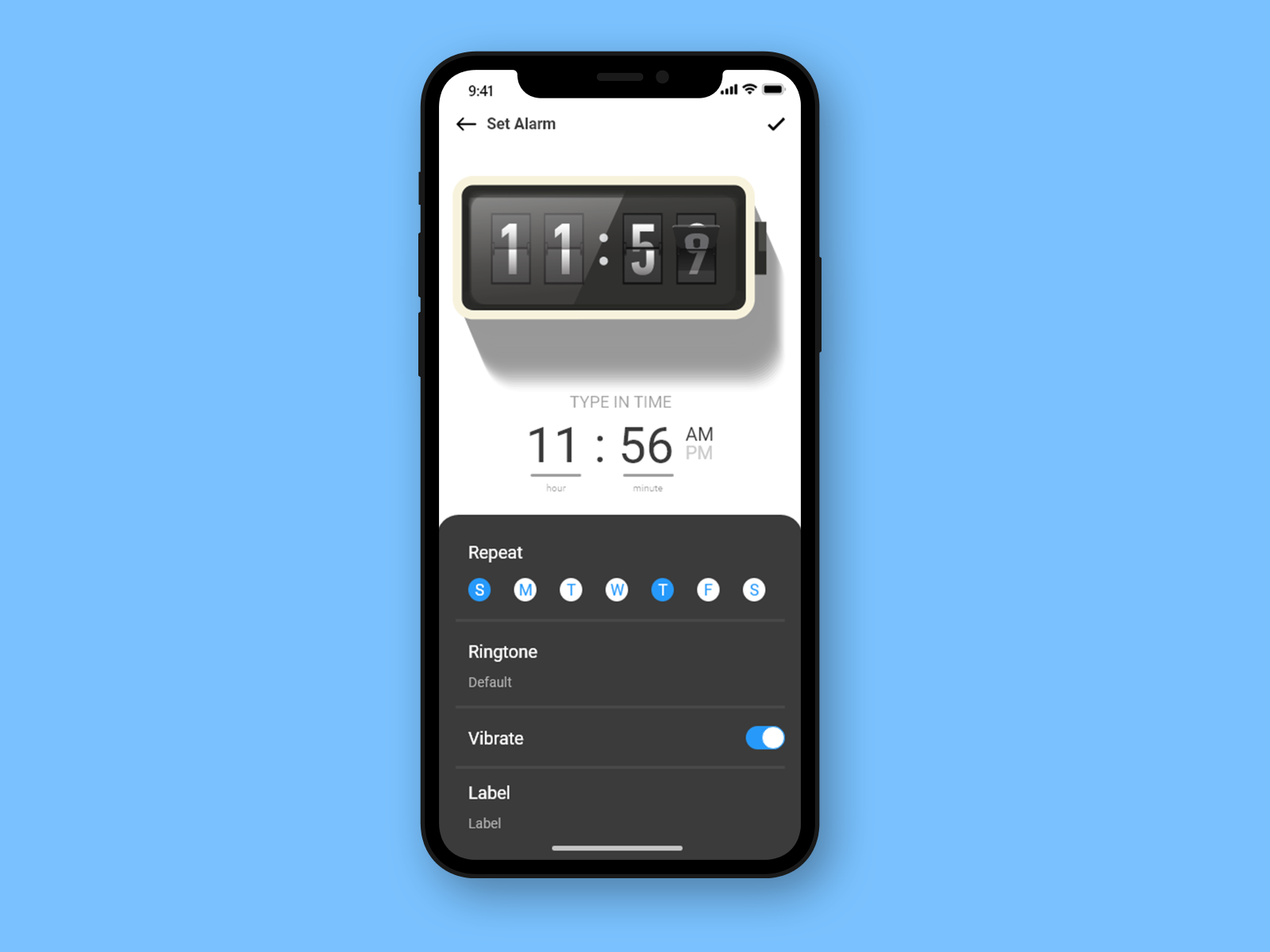The image depicts a conceptual screenshot of an iPhone screen displaying the alarm setup interface. The primary background is a blue rectangular box, within which is the iPhone screenshot.

At the top of the iPhone screen, the status bar shows a time of 9:41 AM, full cellular reception bars, full Wi-Fi signal, and a battery level of 100%.

Below the status bar, there's a navigation header with the label "Set Alarm," accompanied by a back arrow on the left and a checkbox on the right. Directly beneath this header, there is an image of a digital alarm clock with a shadow effect, displaying the time 11:59 AM. The clock appears to be in the process of flipping to 12:00.

Further down, the interface includes a field labeled "Type In Time," with the currently typed time set to 11:56 AM.

Following this, there's a modification section starting with "Repeat," showing the abbreviated days of the week (S M T W T F S), with Sunday (S) and Thursday (T) filled in to indicate the alarm will repeat on these days.

Next is the "Ringtone" option, with "Default" selected. Below the ringtone option is a "Vibrate" toggle switch, which is turned on.

Finally, at the bottom of the screen, there's a "Label" section with the word "Label" currently selected as the label name for the alarm.